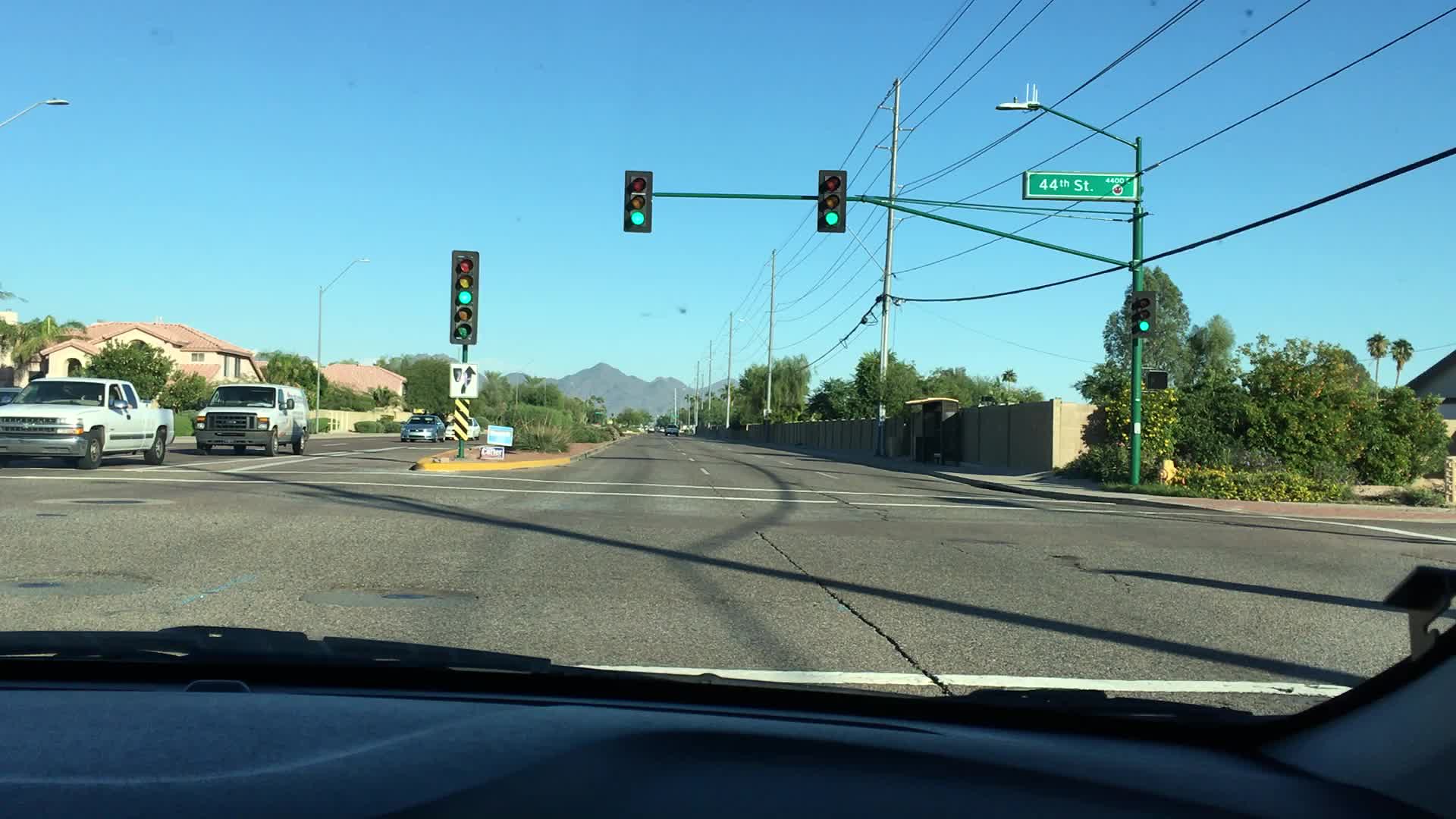A color photograph captures an expansive American road from the vantage point of the passenger seat, looking through the windshield. The wide road accommodates vehicles traveling on the right-hand carriageway; a white pickup truck, a white van, a silver car, and a white car are visible on the left-hand carriageway. Above the road, a network of overhead cables stretches out, connected to green light poles with attached traffic lights, which are currently green. Shadows of these cables and traffic lights are cast onto the sunlit pavement, emphasizing the clear blue sky devoid of clouds. A street sign indicating "44th Street" is prominently displayed. In the distance, a range of rocky mountains looms, accompanied by stone-built houses and clusters of trees. The photograph also includes minor details like the front dash of the car and part of the windshield wiper, adding to the realism of the image. This scene, rich with both natural and man-made elements, appears to capture a moment of tranquility on a bright, sunny day.